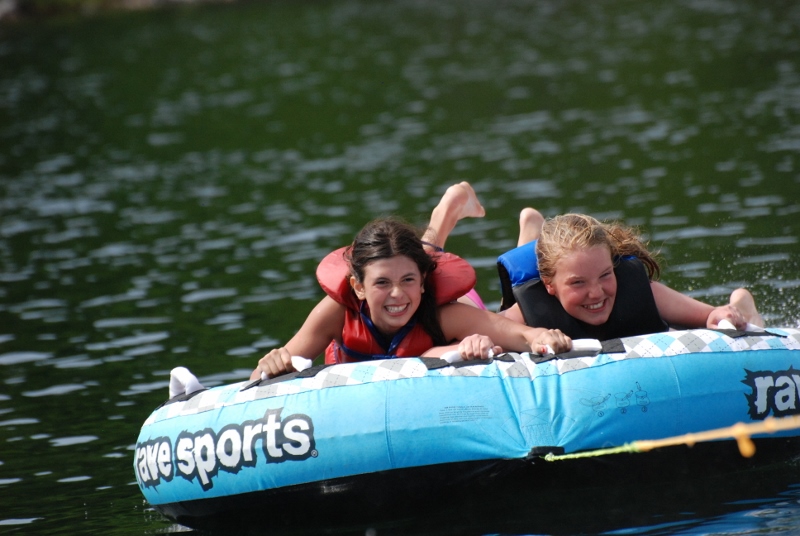In this captivating image, two young girls are enjoying a thrilling ride on a blue, white, gray, and black inflatable raft labeled "Rave Sports" in bold letters. Pulled by a yellow rope, possibly attached to a speedboat, they glide across the green water of what appears to be a lake or river on a bright, sunny day. The girl on the left, a white female with dark hair, is clad in a red life jacket, while her companion on the right, also white with blonde hair, wears a blue and black life jacket. Both girls are gripping the handholds on the raft tightly to keep from falling off, their feet lifted in the air from the motion, reflecting their exhilaration and joy as they have the time of their lives. They seem utterly engrossed in their adventure, not looking directly at the camera, but their radiant expressions perfectly capture the fun and excitement of their waterborne escapade.